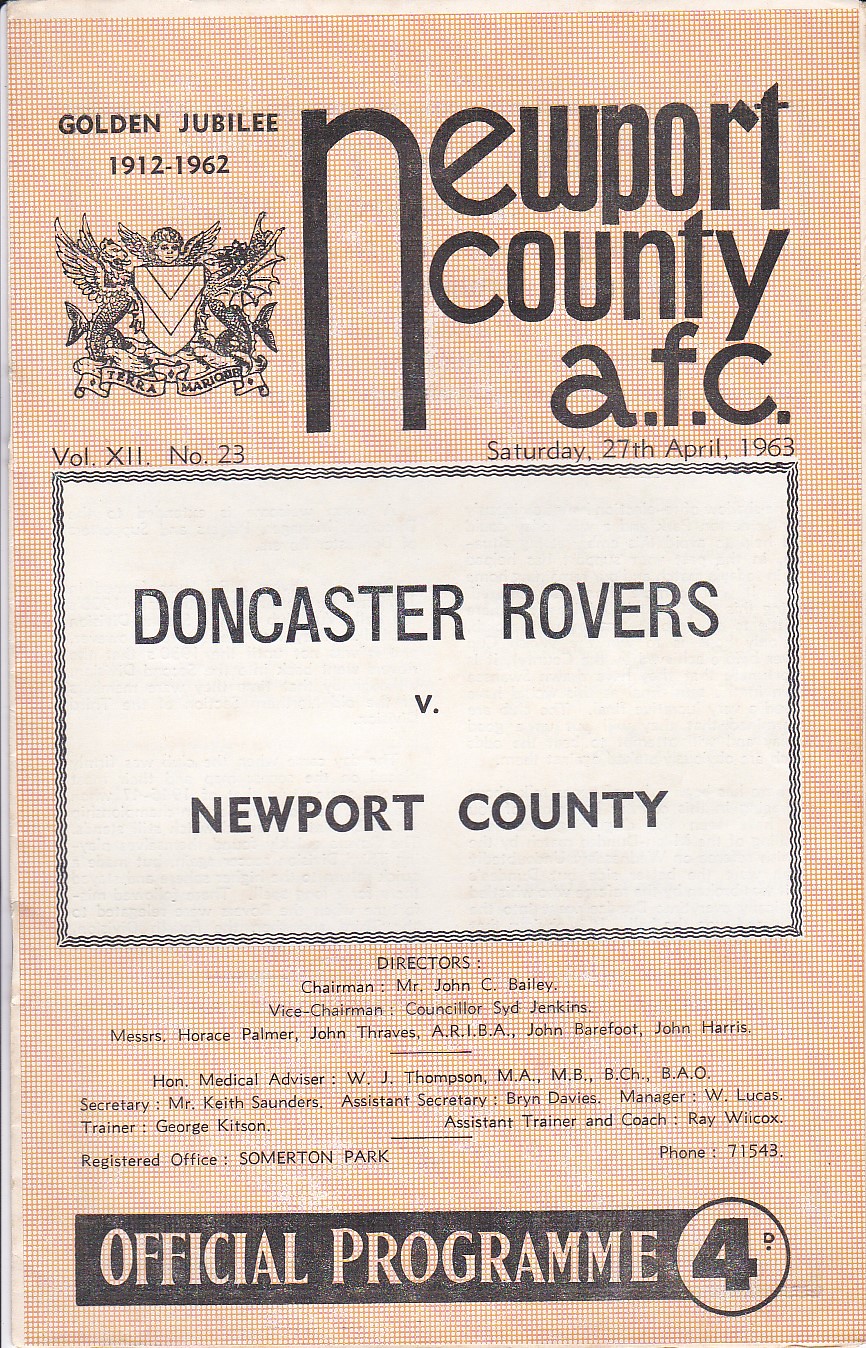This is an image of an official sports program for a football match, featuring a beige cover with black lettering. The program commemorates the Golden Jubilee (1912-1962) of Newport County AFC and is dated Saturday, 27th April 1963, volume XII, number 23. The cover prominently displays a logo on the left side that partially shows an angel with wings and a guard, along with a crest coat of arms. The center text announces the match between Doncaster Rovers and Newport County. Below this, there is a list of directors and other officials associated with the team. The program is marked as the official documentation for this event, highlighting the historical significance and long-standing heritage of Newport County AFC.